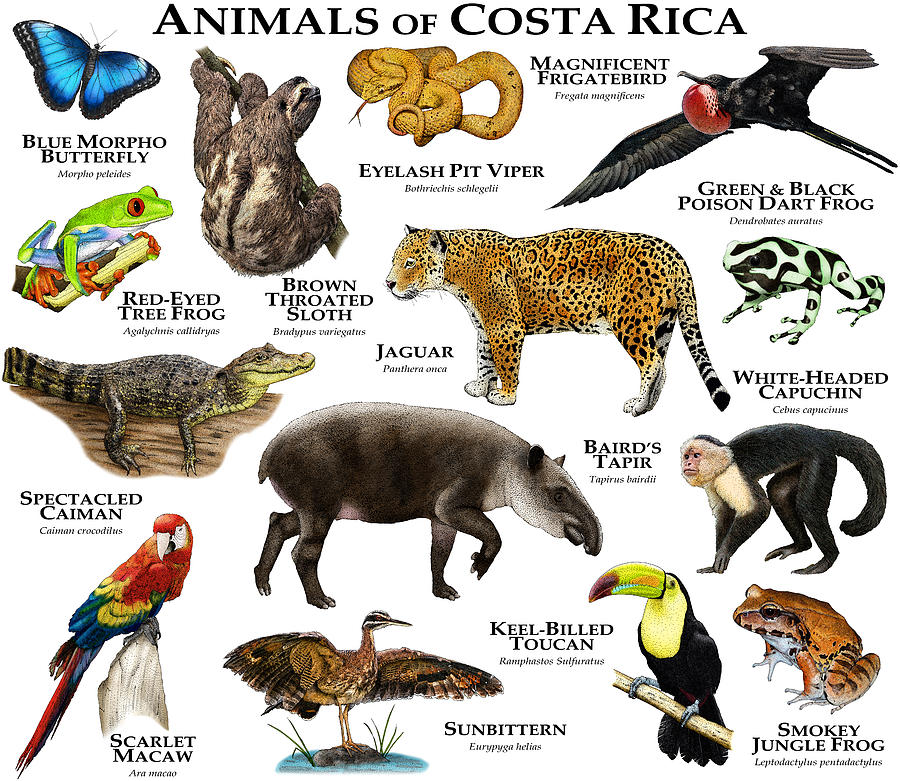The white-background poster, titled "Animals of Costa Rica," features detailed illustrations and the scientific names of various native animals. Starting from the top, the poster showcases a blue morpho butterfly with vivid blue wings bordered in black, followed by a brown-throated sloth hanging from a tree branch. Next is the gold-hued eyelash pit viper. The magnificent frigatebird, distinguished by its black feathers and red neck, is also included. Additional animals depicted are the vibrant red-eyed tree frog, the elusive jaguar, the green-and-black poison dart frog, and a spectacled caiman resembling an alligator. The Baird's tapir, white-headed capuchin monkey, colorful scarlet macaw, long-legged sun bittern, keel-billed toucan, and smoky jungle frog complete the list. Each animal is accompanied by its picture and scientific name, offering a comprehensive visual guide to the rich biodiversity of Costa Rica.